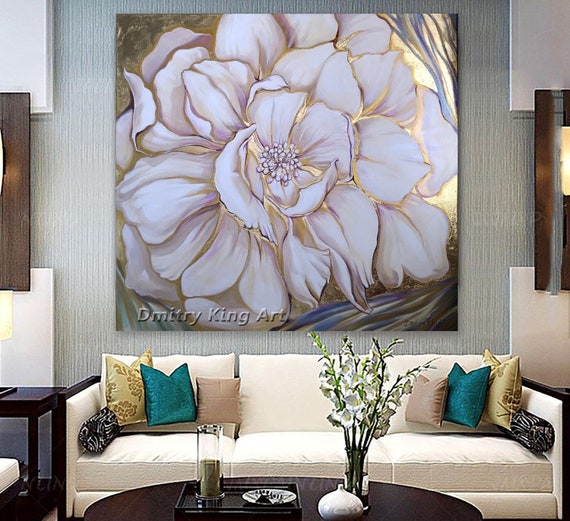This image showcases an elegantly decorated room that might be part of a curated display or someone's sophisticated home. Dominating the center of the image is a striking square painting featuring a pristine white rose or a similar white flower, set against a luxurious gold backdrop. The artwork, which prominently bears the signature "Dimitri King Art" in the bottom left corner, serves as a focal point of the room.

In front of the captivating piece, a comfortable tannish-white sofa is adorned with an array of decorative pillows in varying hues of gold, teal, and reddish-brown. In front of the sofa, a sleek black table holds a small glass vase with fresh flowers, a candle, and a few other decorative items on a black tray, contributing to the room's inviting ambiance. Additionally, a matching black side table is positioned next to the sofa, further enhancing the room's cohesive and stylish design.